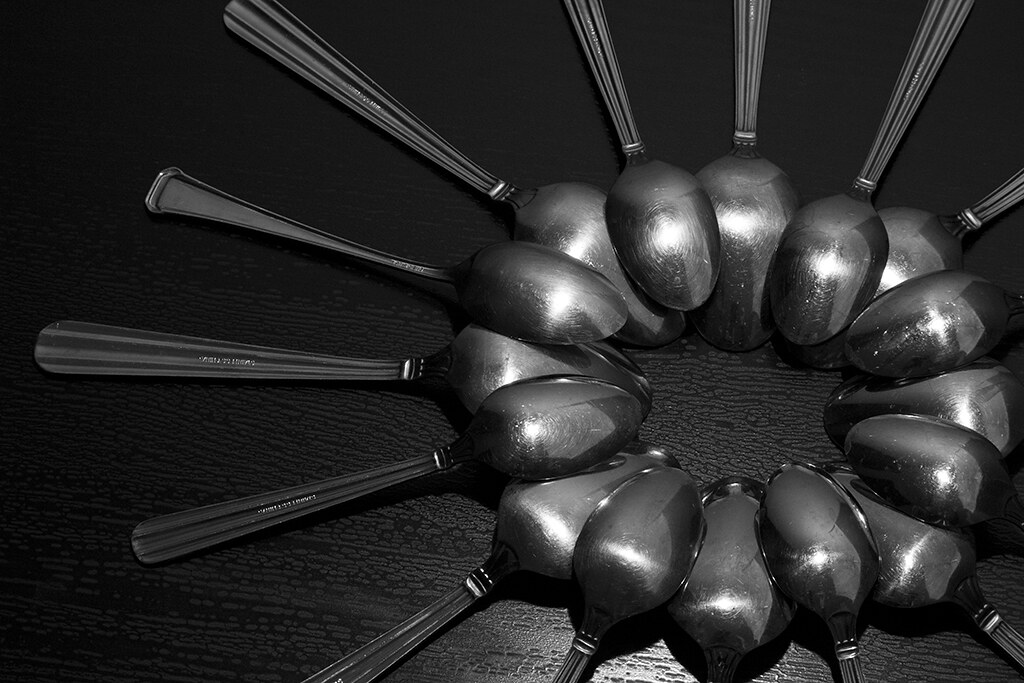This striking black-and-white conceptual photograph presents an array of stainless steel spoons arranged in a sunburst or radiant flower pattern. Positioned slightly towards the bottom right of the frame, the spoons are laid with their concave parts facing downwards, creating a reflective, intricate circle that appears to glow subtly under a specific light source. The spoons vary in handle design—some ending in flat, rounded tips, others longer, wider, or adorned with striations. Though not perfect or symmetrically placed, the spoons interlay atop one another, forming a captivating, asymmetrical composition that blends chaos and artistry. The background at the top is a deep black, devoid of detail due to insufficient lighting, while the lower portion reveals a highly varnished wooden surface, subtly visible with a noticeable grain texture. Some spoon handles, particularly on the left, carry small, unreadable writing, enhancing the detailed complexity of the arrangement. Overall, the photograph's mastery lies in its ability to transform everyday objects into a compelling, almost abstract piece of art.